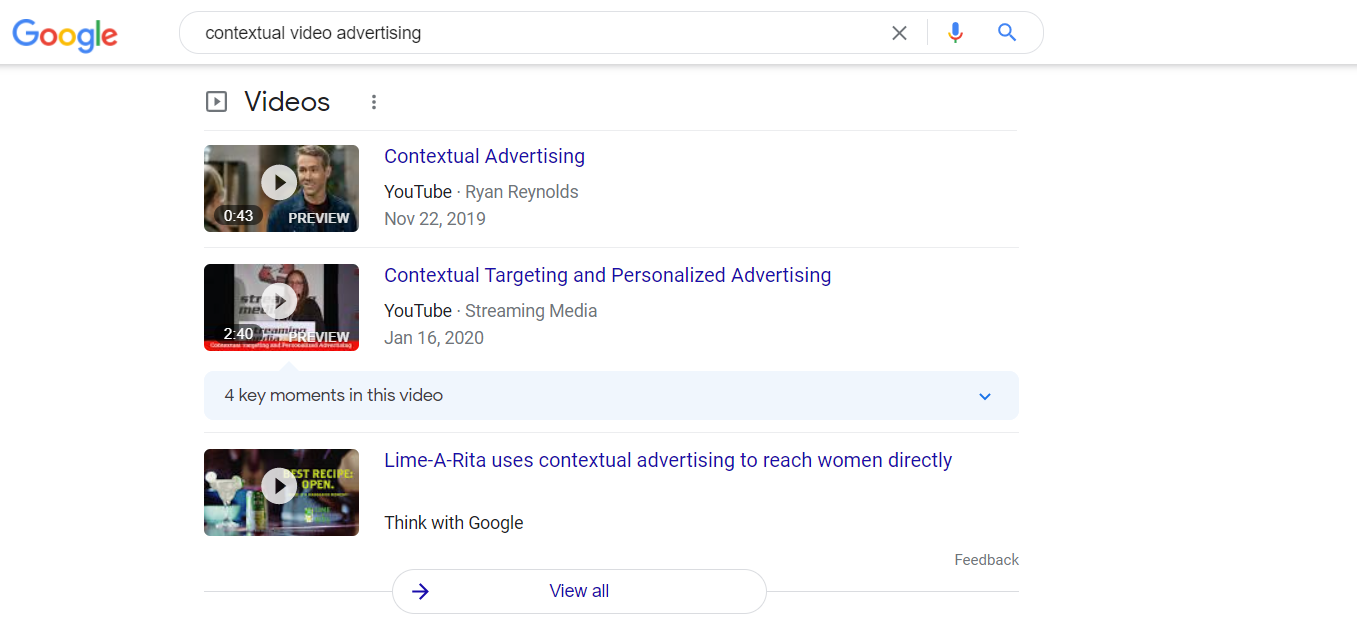The image showcases a Google video search interface with the search query "contextual video advertising" typed into the search bar. At the top of the interface, the recognizable Google logo is prominently displayed, followed by the search bar housing the text. Within the search bar, situated on the left, are three icons: an 'X' icon for clearing the search, a microphone icon for voice input, and a magnifying glass icon for initiating the search. 

Directly below the search bar, the label "video" is visible, accompanied by a box with a play arrow symbol to its right. Beneath this section, three video results are listed. Each video entry includes a thumbnail image on the right side and corresponding titles on the left. The titles of the videos are as follows: "Contextual Advertising," "Contextual Targeting and Personalized Advertising," and "Lime-A-Rita Uses Contextual Advertising to Reach Women Daily."